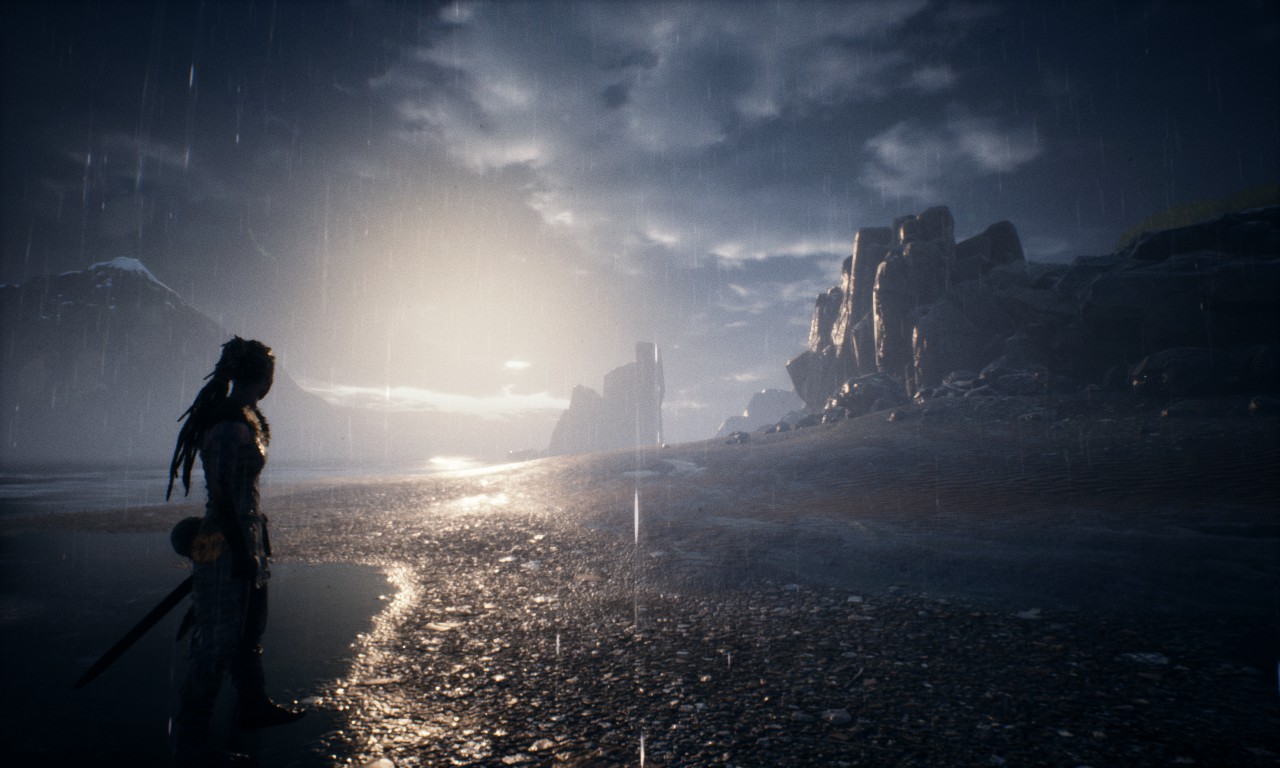This evocative image layers a multitude of details within a dark, atmospheric setting. Dominated by a moody sky filled with thick, ominous clouds, the scene captures the brief, dramatic light of either sunrise or sunset piercing through. It appears to be raining, adding a further layer of depth and texture. Central to the composition is the silhouette of a woman with long hair that reaches down to her mid-back. She is emerging from the ocean, standing at the boundary where the deep, dark blue of the water meets a beach strewn with shells and small pebbles. There is a sword hanging from her left side, suggesting an element of mysticism or fantasy. The woman, outfitted in what could be a crop top and long pants, gazes forward toward the horizon, where massive rock formations rise alongside what might be distant buildings on a hill. The overall ambiance of the image, which perhaps belongs to a video game or a detailed painting, evokes a sense of isolation and intrigue heightened by the dark tones and the interplay of natural and surreal elements.